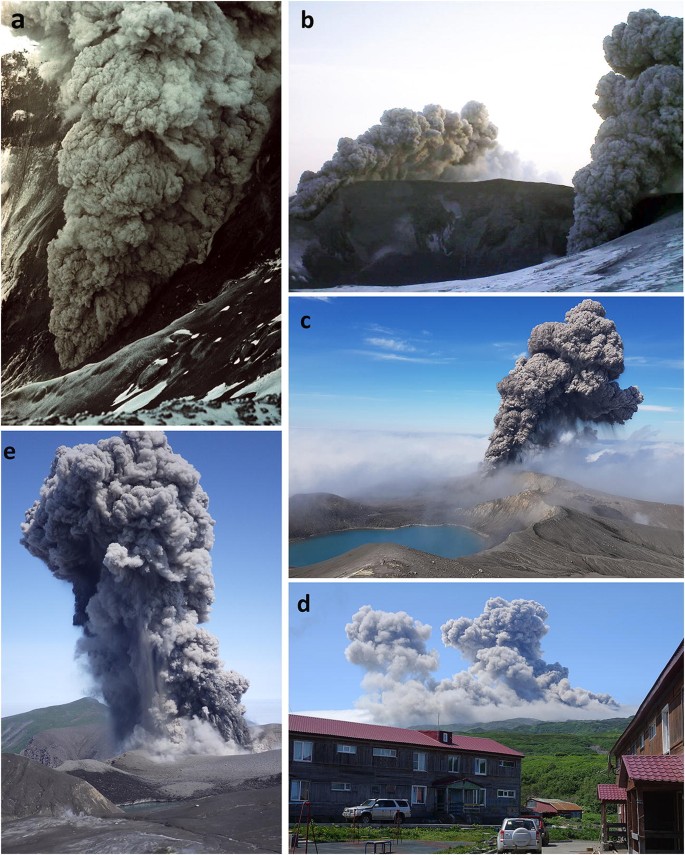The collage features five distinct images of a volcanic eruption, labeled A, B, C, D, and E, offering various perspectives of the dramatic event. 

Image A, located in the upper left corner, provides a close-up view of thick, dark gray plumes of smoke billowing skyward, set against a backdrop of volcanic rock. The composition offers no visible landscape or lava flow, focusing primarily on the dense smoke. 

Image B, situated in the upper right corner, zooms out slightly to reveal a split view of sky and volcanic crater, capturing multiple sections of smoke plumes rising from different sources. This photograph offers a broader perspective, with around 30% of the frame covered in smoke and the other half dominated by a clear sky.

Image C, positioned in the middle right, presents an even wider aerial shot, showcasing not only the volcanic crater and smoke plumes but also a large, bright blue lake below and to the left of the eruption. The desolate, rocky landscape contrasts with the vivid blue of the sky and water, highlighting the magnitude of the eruption.

Image D, found at the bottom right, features a landscape with visible human elements: two brown wooden buildings with red roofs, several cars, and a playground in the foreground. The background depicts green valleys, trees, and the volcanic ridge, with huge smoke plumes dominating the sky.

Image E, located in the bottom left corner, captures another close-up of the eruption, emphasizing the powerful, thick smoke and debris thrusting upwards. The background reveals hints of a green mountain ridge and possibly the edge of the lake, though the focus remains on the smoke which occupies about 70% of the frame.

The photographs are arranged with A and E being vertical on the left, and B, C, and D as horizontal images on the right, providing a comprehensive and striking visual narrative of the volcanic eruption from multiple angles and distances.